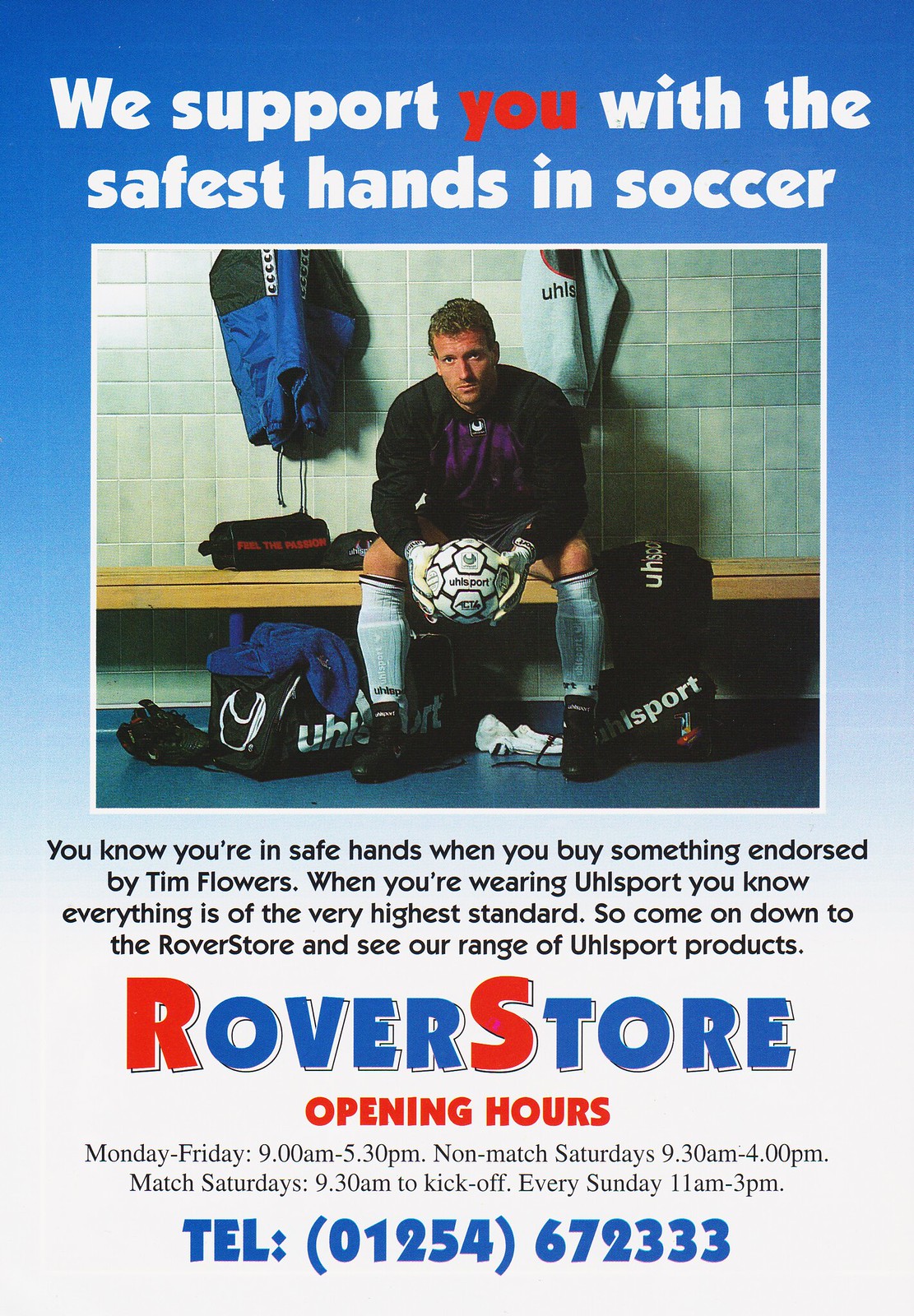The poster is an advertisement for Rover Store, prominently featuring the title "We Support You With The Safest Hands In Soccer." The upper part of the image has a blue background with the word "you" printed in red, and the rest of the title in white text. Below the title, the poster showcases a man, presumably soccer player Tim Flowers, seated on a wooden bench in front of a green-tile wall, suggesting a gym locker room setting. He is donning a black and purple jersey paired with white shorts and holds a white soccer ball adorned with red lines and patterns. To the left on the wall, a green and black coat is hung, while a white T-shirt hangs to the right. 

The narrative continues with details about Rover Store, emphasizing their high-standard sports products, including Tim Flowers' YuleSport brand. The store's opening hours are listed: Monday to Friday from 9 am to 5:30 pm, non-match Saturdays from 9:30 am to 4 pm, match-day Saturdays from 9:30 am until kick-off, and Sundays from 11:30 am to 3 pm. The flyer further includes the store's contact number: 01254 672333.